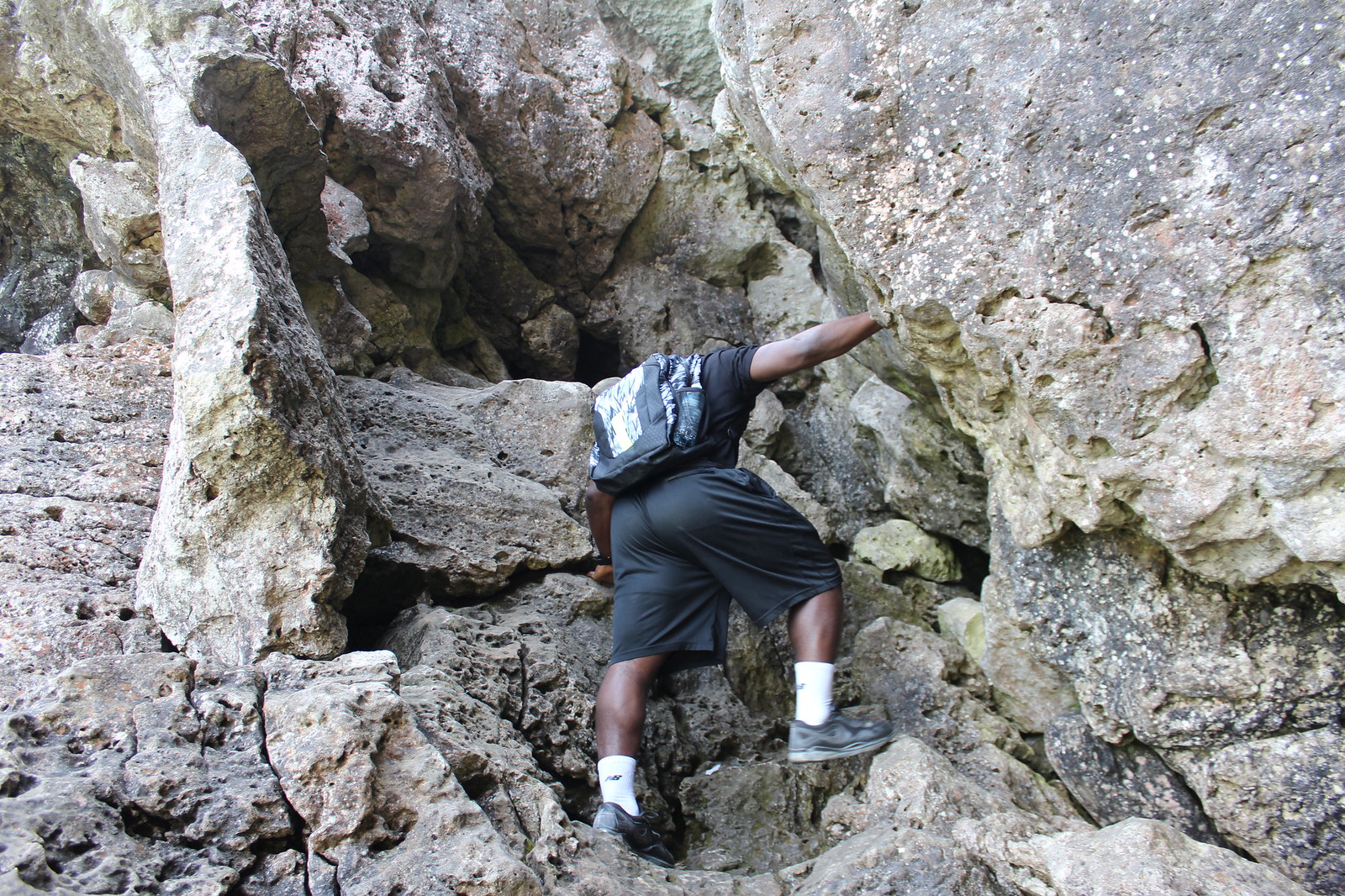The full-color photograph captures an African-American man from behind as he climbs the jagged, gray, rocky surface of a natural cliff or large hill in an outdoor, daytime setting. He is dressed in a black t-shirt, long black shorts, dark tennis shoes with tall white socks, and a backpack that includes a water bottle in its side pocket. The rock face he is scaling appears to be solid rock with no vegetation, suggesting it may not be very tall or requiring specialized climbing gear.